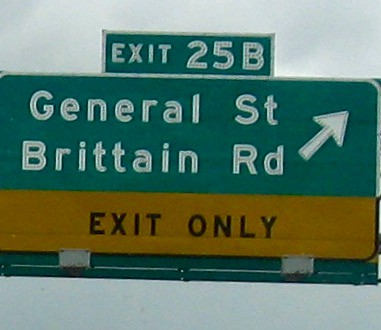This photograph prominently features a large highway street sign consisting of a main rectangular section and a smaller attached rectangle on top. The main sign's upper part has a green background and displays the words "General St" and "Britton Rd" in bold white letters. A diagonal white arrow pointing northeast is also visible, indicating the direction of these roads. Below this, a yellow section within the main rectangle states "EXIT ONLY" in black letters. Above the main sign, the smaller rectangular sign reads "EXIT 25B" against a green background with white text. The photo captures a hazy sky in the backdrop, partially obscuring the signs.